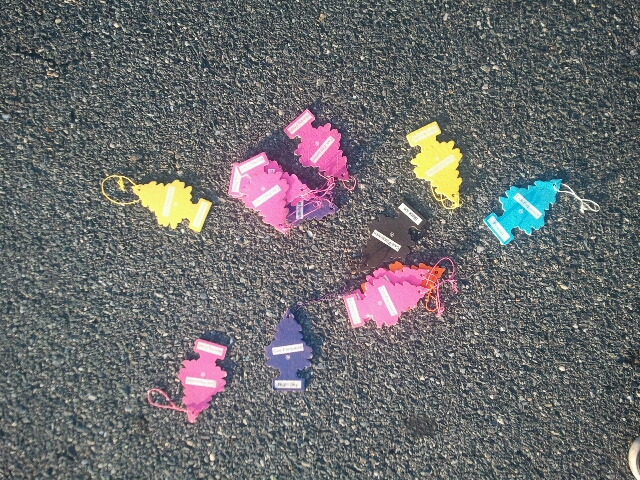The image is an overhead photograph taken on black-gray asphalt, likely in a parking lot or on a road. Scattered across the pavement are 13 tree-shaped car air fresheners, known as "Little Trees," each displaying a variety of colors: several pinks, two yellows, one light blue, one purple, one orange, and one black. The air fresheners, each approximately 4-5 inches tall, are positioned randomly, with some upright and others upside down, revealing the strings used to hang them, typically from a car's rearview mirror. The photo, while bright, is somewhat blurred and amateurish, with a hint of a shoe visible in the bottom right corner. The labels on the air fresheners are too small to read, and the entire scene is centered on the asphalt background.